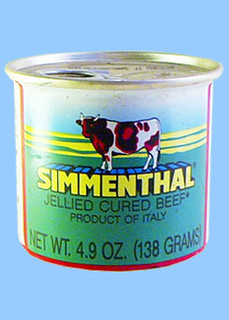The image depicts a close-up of a can of "Simmenthal Gelled Cured Beef". The can itself has a shiny silver metal top with a pull-ring for easy opening. The label design features a light blue sky-like upper section transitioning to green at the bottom. Encircling the label is a red outline with additional white along the sides, giving it a framed appearance. Prominently centered on the label is an illustrated cow with a red, brown, and white coat, and white horns, standing in front of three yellow lines. Just above the cow is the brand name "Simmenthal" in thick yellow letters. Beneath it, in black text, are the words "Gelled Cured Beef" followed by "Product of Italy". Further down, the net weight is specified as "Net Weight 4.9 oz (138 grams)". The comprehensive details and colors, such as the blue and green sections along with red and white borders, create a visually appealing and informative package design.